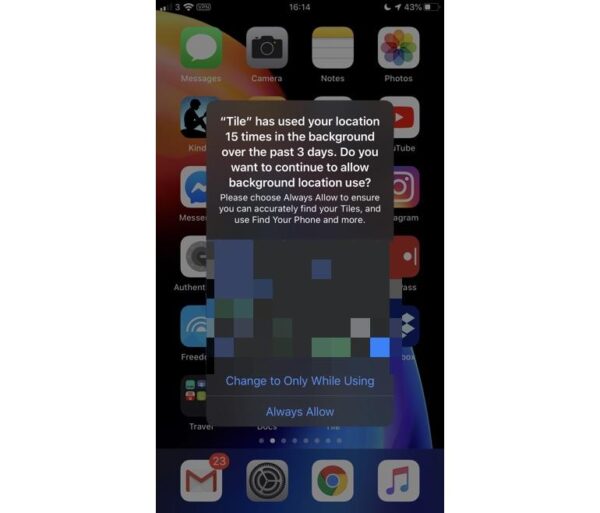A smartphone is displayed, showcasing a detailed and vibrant home screen. The screen indicates a full Wi-Fi signal and a battery level at 614%, represented with a half-moon icon. A location chart showing 643% is also present. Dominating the view is a green square labeled "Messages" alongside a variety of app icons including Camera, Notes, Photos, and Kindle (represented by a person icon). Additional icons for YouTube, Instagram (depicted with a purple background and white lines), Authenticator, Freedom, and Java are visible. 

In the bottom left corner, the screen includes icons for Gmail, Settings, and Google Chrome. The music app is prominently displayed with a background featuring purple and black hues, accompanied by scattered grey and white dots.

A notification tile is highlighted, indicating a recent message from the Tile app. The notification states: "Tile has issued a request for 15 tiles in the background for the past few days. To continue allowing background location access, ensure the setting is set to always allow to locate tiles and use them to find your phone or other items. If permissions have changed, adjust to 'Only while using' or 'Always allow' accordingly."

This organized and detailed arrangement on the smartphone's home screen provides a clear and functional interface for the user.